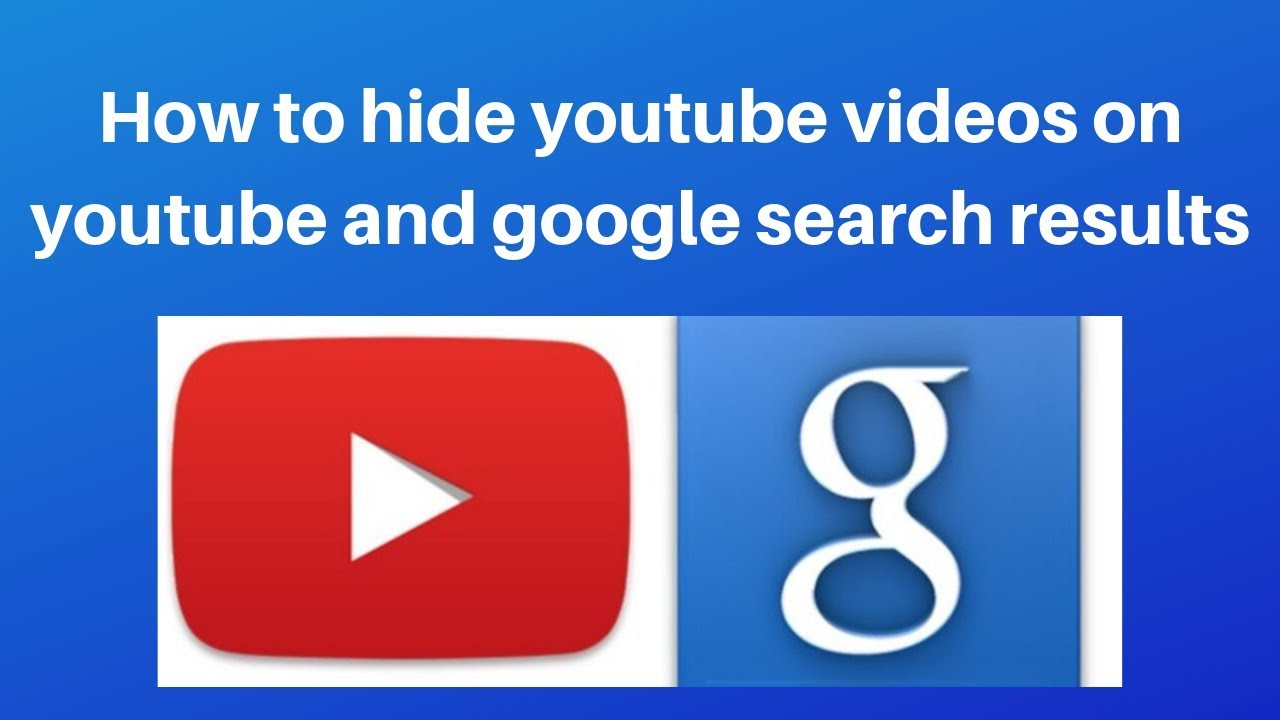This image features a predominantly blue background with a white strip at one end. Overlaid on the background is white text that reads, "How to Hide YouTube Videos on YouTube and Google Search Results." Centrally positioned on the blue backdrop is a large white rectangular box, which gradually transitions into blue at one end. Inside this box, there is a notable red square containing a white right-pointing arrow, symbolizing YouTube. Adjacent to the red square is a smaller blue square with a white lowercase "g" inside, representing Google. This organized layout visually conveys the steps and tools required for hiding YouTube videos from both YouTube and Google search results.